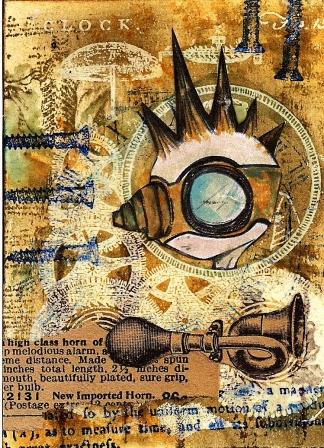The image appears to be a vintage-themed artwork, characterized by a hodgepodge of various elements layered upon a background resembling old, brownish paper. Central to the composition is a white illustration of a child with a mohawk, donning goggles with a nosepiece. Surrounding this figure, the artwork features a mixture of sepia-toned designs, such as a horn and white circular patterns that evoke the appearance of lace or gears. Additional details include black or blue screws printed over the layers, along with intricate, faded patterns that enhance the antique feel of the piece.

In the top section of the image, there is a war clock, and nearby, some spikes and what appears to be a glass or magnifying glass add to the eclectic mix of visuals. The overall aesthetic is reminiscent of a comic book illustration, with images of nails and various other motifs scattered throughout. 

Text is interspersed within the piece, giving it a collage-like quality. Phrases like "high-class horn of melodious alarm" can be discerned to the left of the horn, although the full text is often fragmented. Further readable snippets include "distance made," "total length two and a half inches," "die mouth beautifully plated shear grip," "bulb 2131 new imported horn," and partially obscured sentences like "postage and some other," "uniform motion," and "measure time as a."

The entire composition, tinted in golden brown hues, evokes the ambiance of a bygone era, akin to a vintage treasure map or a poster advertising museum artifacts.